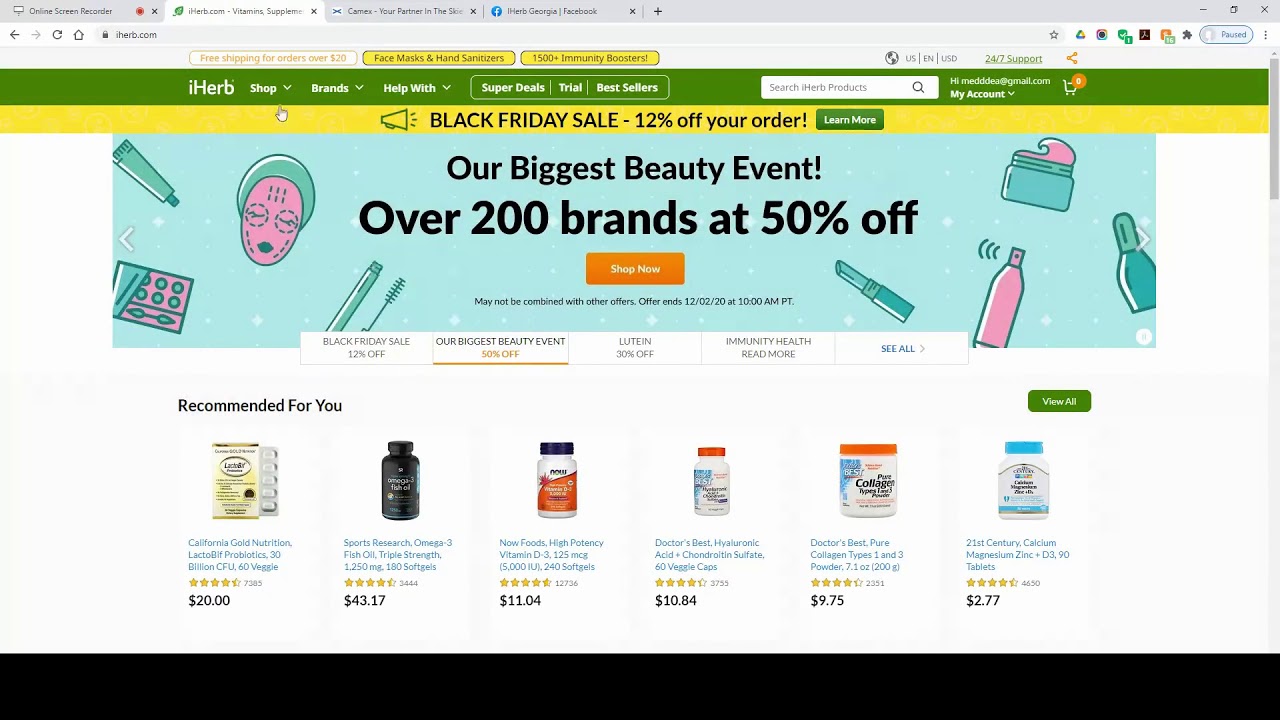The image appears to be a screenshot of a web browser, likely Google Chrome or Microsoft Edge, displaying the iHerb website. The website features green branding with a green search bar at the very top. A prominent banner announces "Black Friday Sales" with a 4% discount on orders. Below the banner, there's a hero section highlighting the message, "Our Biggest Beauty Event: Over 200 Brands at 50% Off." There is also a "Shop Now" button included in this section.

Next to the left and right sides of the main content, there are additional promotional slides indicating various offers: "Black Friday Sales - 20% Off," "Our Biggest Beauty Event - 50% Off," "Lutein - 30% Off," and categories like "Immunity," "Health," and "Brain." There is also an option to "See All" these offers.

A recommendation row titled "Recommended For You" displays various products including:
- California Gold Nutrition Probiotics
- Source Naturals Omega-3 Fish Oil
- Triple Strength Fish Oil
- NOW Foods Vitamin D
- Ascorbic Acid
- Chlorella Sulfate
- Pure Collagen Types I and II
- 21st Century Calcium, Magnesium, Zinc, and Vitamin D3

This detailed setup aims to encourage purchasing decisions during the promotional event.